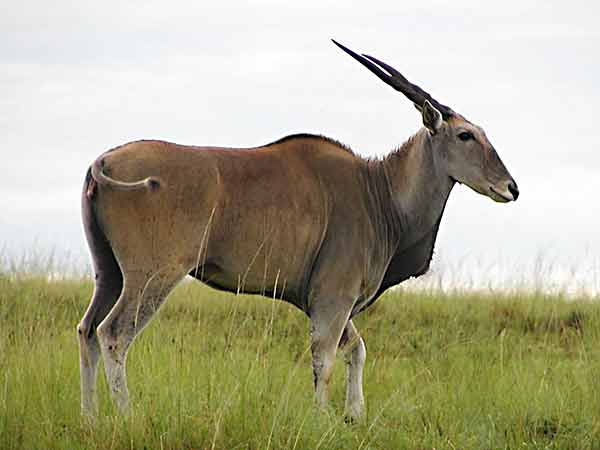This horizontally oriented outdoor photograph captures a majestic impala standing amidst tall green grasses in the wild. The impala, an African antelope, exhibits a robust body that's predominantly brown with light grayish-brown legs and head. Its long, straight, and slightly spiraled black horns curve elegantly backward from its forehead. The impala features a mild hump on its back and a small, unadorned tail with a tuft of hair at the end, which it appears to be swishing. Its neck, slightly protruding before angling sharply back into the body, supports a long, narrow, and triangular head aligned straightforward, suggesting calmness and a healthy disposition. The impala stands unperturbed in the grassland, offering a serene view of its prominent and distinctive features against the lush, green backdrop.